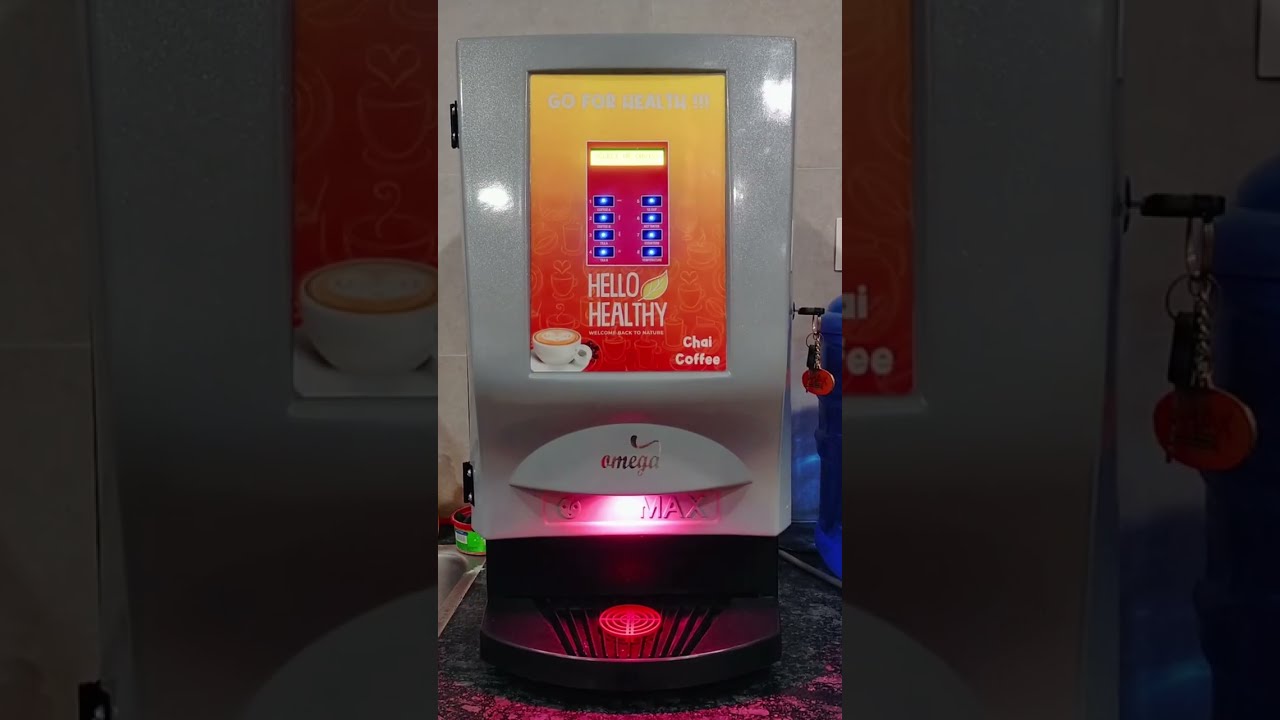The image depicts a detailed view of a coffee dispensing machine or coffee maker situated on a sleek black countertop to the right of a sink. This sophisticated machine features a black base and a silver body, which houses a prominent display screen at its center. The screen showcases a vibrant yellow and orange background with the welcoming message "Hello, Healthy" accompanied by a distinctive leaf logo on its right. On the lower half of the screen, to the bottom left, there's a graphic of a white coffee cup, while the bottom right reads "Chai Coffee." Notably, the machine appears to include a key with a keychain hanging from the right side, suggesting it can be unlocked, possibly for maintenance or refilling purposes. The screen is embedded within a border, and the area underneath it appears to glow red, indicating the spot where users place their cups to receive their hot beverage. The machine’s brand, Omega, is subtly incorporated into the design, reinforcing its polished and professional appearance, likely indicative of a business setting.